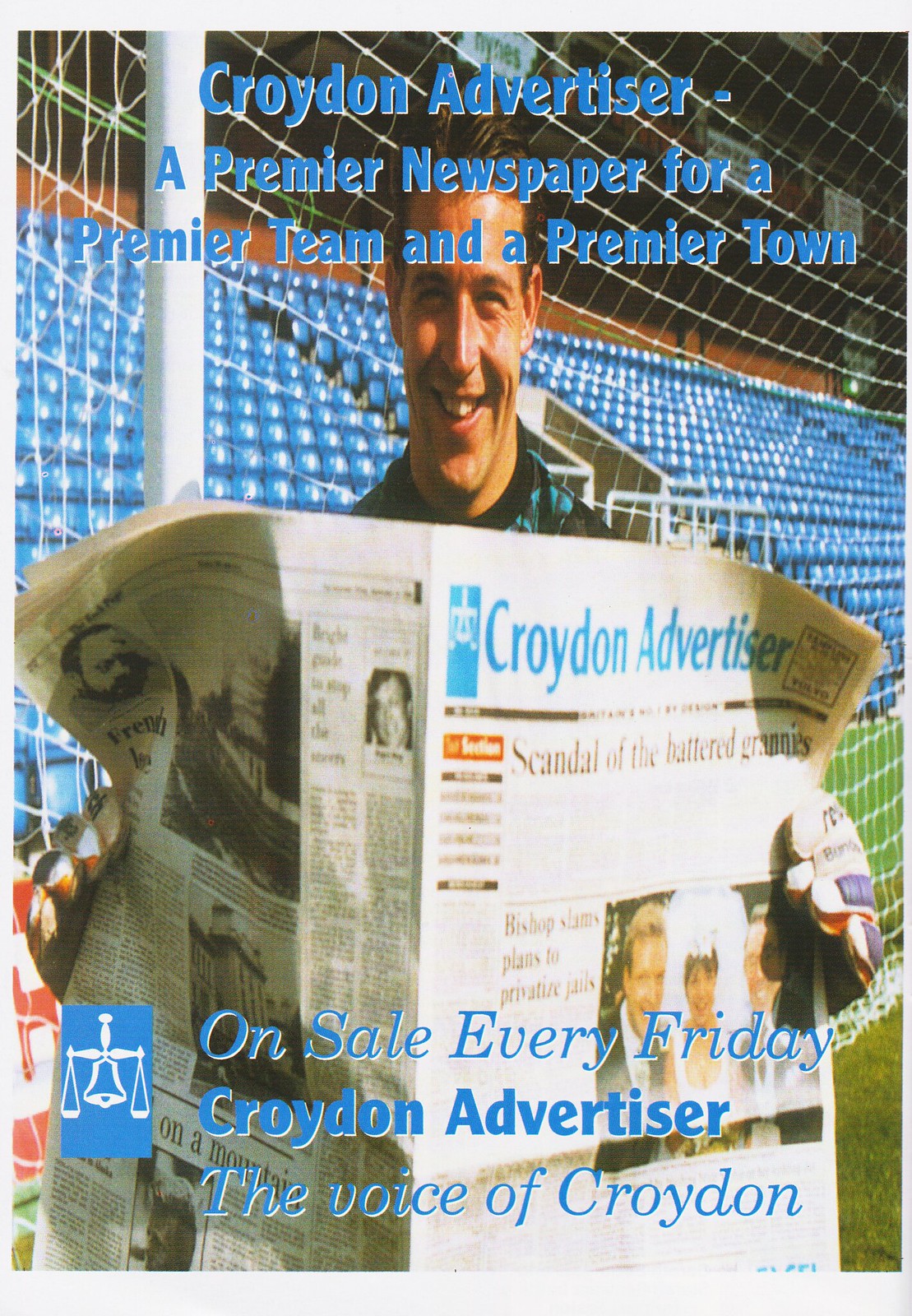The image portrays a white male with brown hair, smiling as he stands outdoors on a football pitch. He is wearing a blue and black jersey and holding a newspaper titled "Croydon Advertiser" in blue text. The man is positioned in front of a goal with a net and empty stadium seats denoted by blue chairs, suggesting he is likely a soccer player. The newspaper he holds prominently features the headline "Scandal of the Battered Grannies" and a picture of a wedding on its front page. Additional articles and pictures of people and buildings are visible on the left side of the open newspaper. Embedded in the image, in blue text, is the statement "On sale every Friday, Croydon Advertiser, the voice of Croydon," accompanied by a logo of white scales inside a blue rectangle. At the top of the image, the tagline reads, "Croydon Advertiser: A Premier Newspaper, A Premier Team, and A Premier Town."